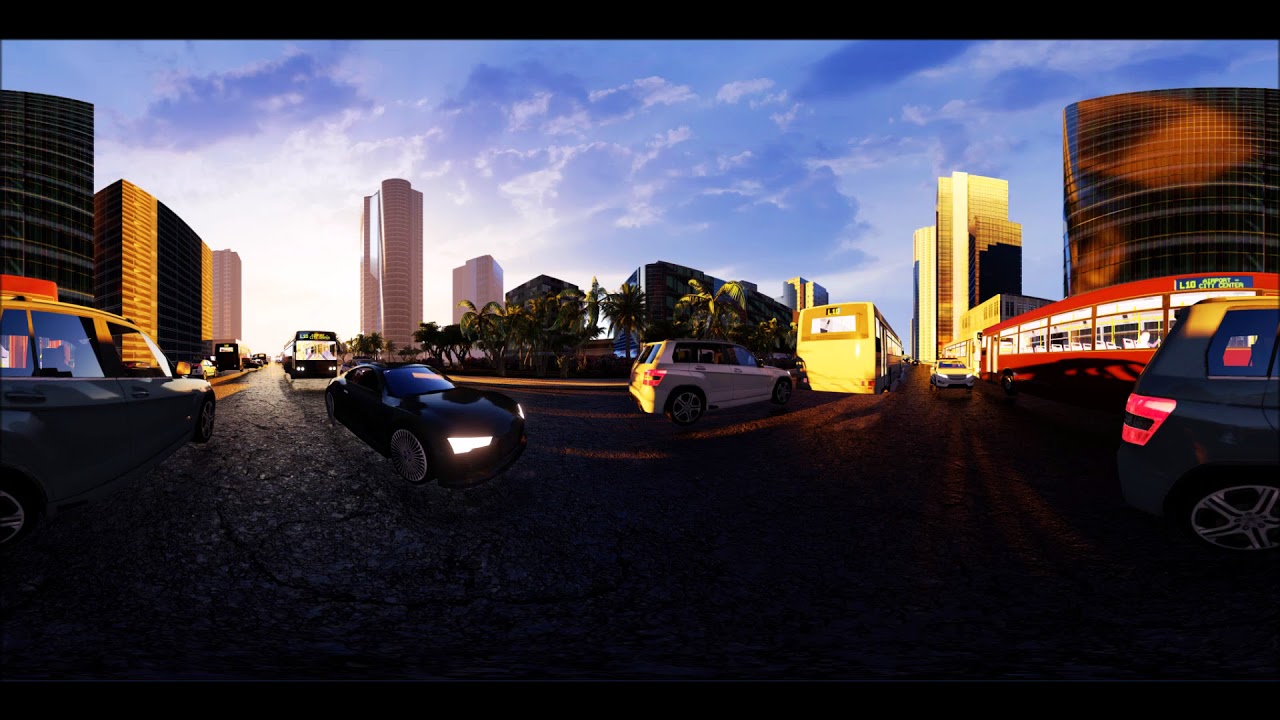The image is a computer-generated, panoramic depiction of a busy city street from a somewhat outdated video game engine. It features a lively urban scene with a dark, gray-brown road that curves around the image. Numerous vehicles, including black sports cars, white station wagons, hatchbacks, and both black and red buses, populate the street. One of the red buses has visible text on its green side, indicating "City Center, L10." The road is divided by a median planted with tropical palm trees, adding a touch of greenery. The cityscape is lined with random high-rises and skyscrapers on the left, center, and right. The sky above is a vibrant blue with splotches of white clouds and is completely white towards the left, transitioning to blue as it ascends, suggesting a sunset setting. The glossy surfaces of some cars reflect the ambient light, enhancing the image's digital aesthetic. The overall scene evokes a bustling Las Vegas vibe, underlined by the game's era-specific textures and details.